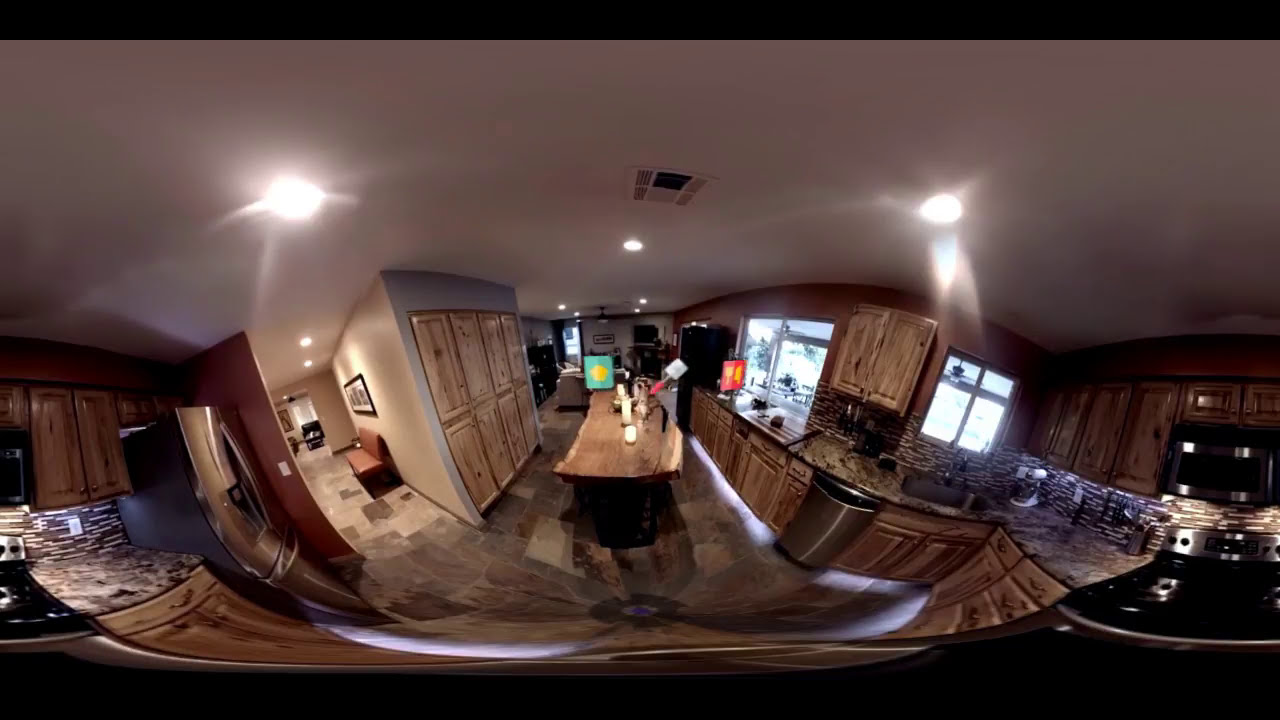The image showcases a modern, panoramic view of a kitchen that combines natural tones with a contemporary design. The scene is busy with detailed elements spread throughout. The camera's curved lens creates a slight distortion, bending the edges and causing objects like the silver refrigerator to appear banana-shaped.

Starting from the left, a hallway with natural stone flooring, predominantly light brown with shades of tan and gray, leads into the kitchen area. A brown leather bench faces left in this hallway. The left wall of the kitchen is dark brown and features a light switch. Adjacent to this is a silver refrigerator and a countertop resembling a zebra print, black and white mix.

A black stove with a microwave above it sits close to the refrigerator on the left. The right side of the hallway displays two rows of four wooden doors, which might be decorative. Further to the right, the kitchen transitions into more countertops and a sink beside a trash can, situated under a window adorned with plants.

In the center of the kitchen, there is a wood island (rectangular in shape) used both for dining and food preparation. This island has various items on it, including some tools like a spatula and possibly candles. The scene is lit by many white ceiling lights, adding to the bright and airy atmosphere.

On the right side of the kitchen, another window above countertops provides more natural light. Further into the background, elements of a living room are visible, including a couch and a TV. The flooring throughout the kitchen and hallway enhances the natural aesthetic with its square stone tiles.

Additionally, artwork and decorative elements enrich the space. There's a painting with a black frame on one wall and a picture with a white background featuring building shapes in the center of view. A green box with a yellow chicken design on it also stands out on the central island, adding a touch of color.

Overall, the kitchen's palette is predominantly brown, with various wood and natural stone textures harmonizing to create a warm, inviting space punctuated by modern appliances and thoughtful decor.